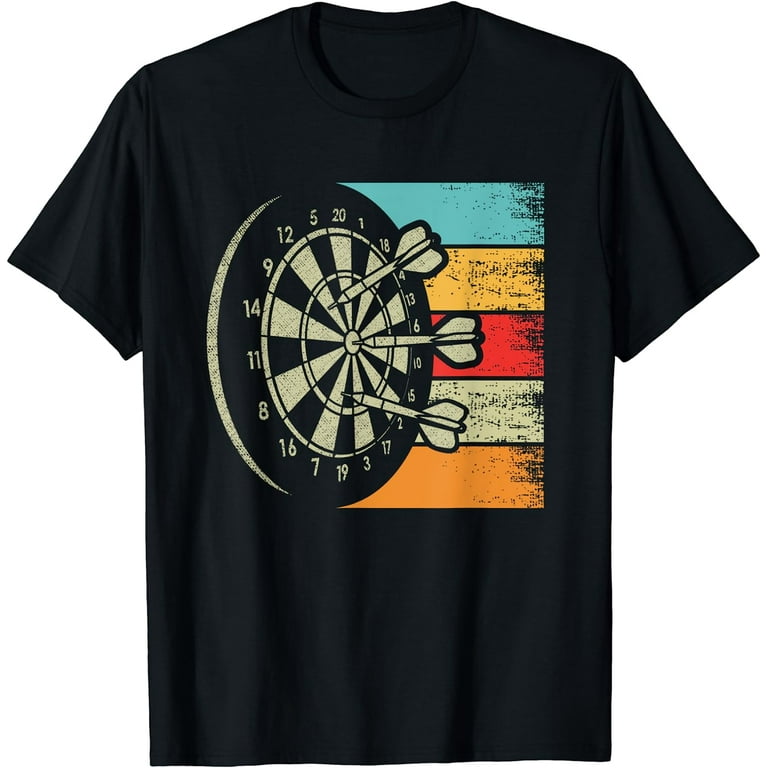The black, short-sleeved shirt, which appears to be designed for men or as a unisex garment, is set against a white or transparent background. Dominating the front of the shirt, approximately two-thirds of the space, is a striking black and white dartboard. This dartboard is detailed with numbers 1 through 20 and features distinct rings signifying different scoring areas. Three darts are depicted on the board, with two embedded in the ring closest to the bullseye and one precisely hitting the bullseye itself. Enhancing the visual appeal, horizontal stripes in vibrant colors – blue, yellow, red, off-white, and orange – form a backdrop to the dartboard. These stripes have a faded, distressed look, adding a stylishly vintage feel without the shirt appearing worn out. The overall design makes for a bold and dynamic statement piece.